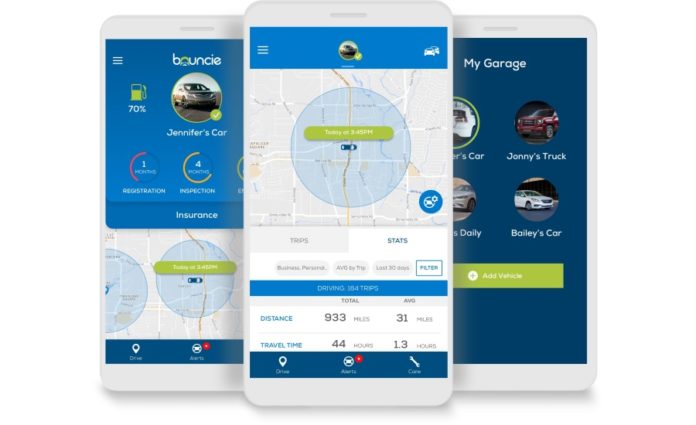The image features a meticulously arranged display of three smartphone prototypes, each encased in sleek silver borders. The central phone screen prominently exhibits a GPS tracking interface, displaying crucial travel metrics such as "Distance" and "Travel Time." To the right, another screen is labeled "My Garage," showing an array of car images accompanied by different people's names, likely representing user profiles or saved vehicles. The leftmost phone screen bears the title "Bouncy" at the top, showcasing a car image and what appears to be detailed statistics related to the vehicle. The trio of screens collectively suggests a multifaceted app designed for vehicle tracking, management, and monitoring.